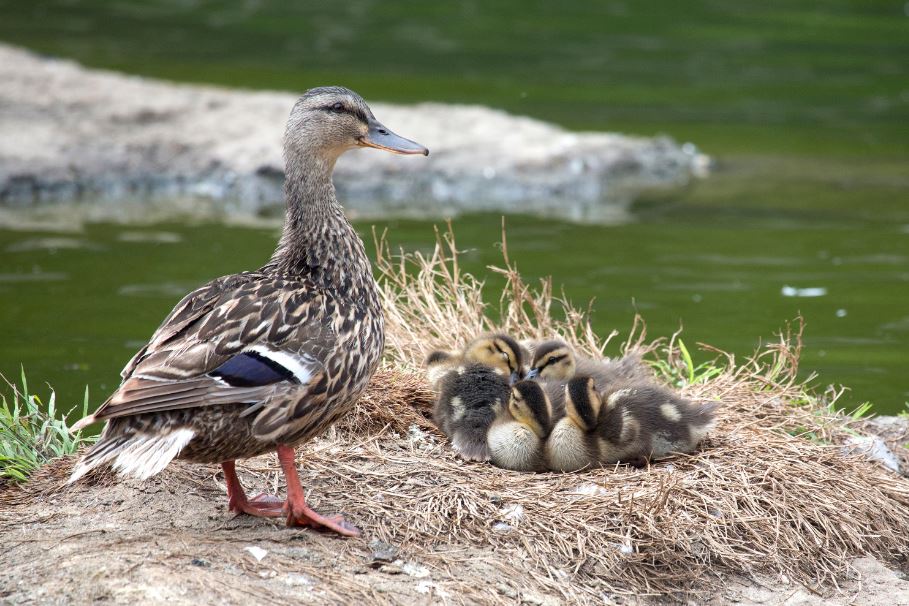A professional daytime nature shot features a serene scene by a green-tinted lake, captured in a square format. The central subjects are a mother duck and her five fluffy ducklings, huddled together in a nest composed of brown brush and fragments of green grass. The mother duck, distinguished by her elegant mix of white, black, grey, and brown feathers, stands protectively over her babies, revealing her red feet and the right side of her face as she looks toward the camera. The ducklings, with their soft downy feathers displaying black and yellow hues, nestle closely in their cozy nest. A mysterious gray object, potentially a rock, log, or even a crocodile, stretches from the upper left across the backdrop, adding an intriguing element to the tranquil scene, which has only minimal background distractions.